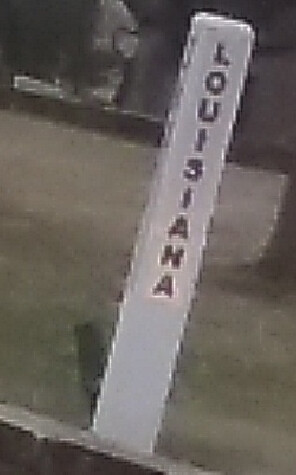This image is characterized by its low resolution and pixelated quality, making it appear very blurry and fuzzy. The photograph has a rectangular shape, and at its center, there is a long, white pole. Along the side of the pole, there is text that reads "LOUISIANA" vertically from top to bottom, written in black. Despite the blurriness, it is possible to discern that the ground in the image has a light brown to grayish hue. Additionally, in the top left corner, there appears to be some indistinct background elements, further contributing to the overall indistinct quality of the image.